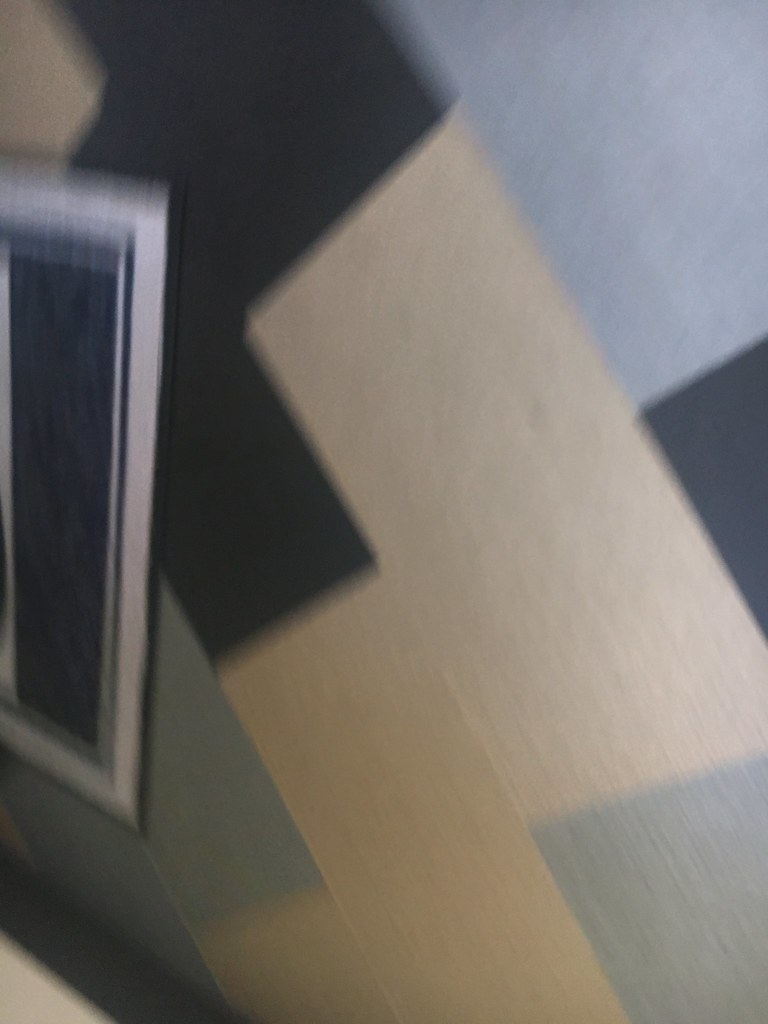This blurry indoor photo captures an overhead view of a patterned carpet with rectangular segments in various colors such as black, gray, light yellowish, tan, light blue, and dark blue. The pattern appears somewhat chaotic, with the rectangles forming a checkered layout, including at least one L-shaped black section. To the left, partially cropped and overlaying the carpet, is another object that resembles either a throw rug or a piece of framed art. It has a black border, a white inner frame, and a dark, indeterminate center. The overall dim lighting and blurred focus add to the ambiguity of the scene. No text or other distinguishing marks are visible.